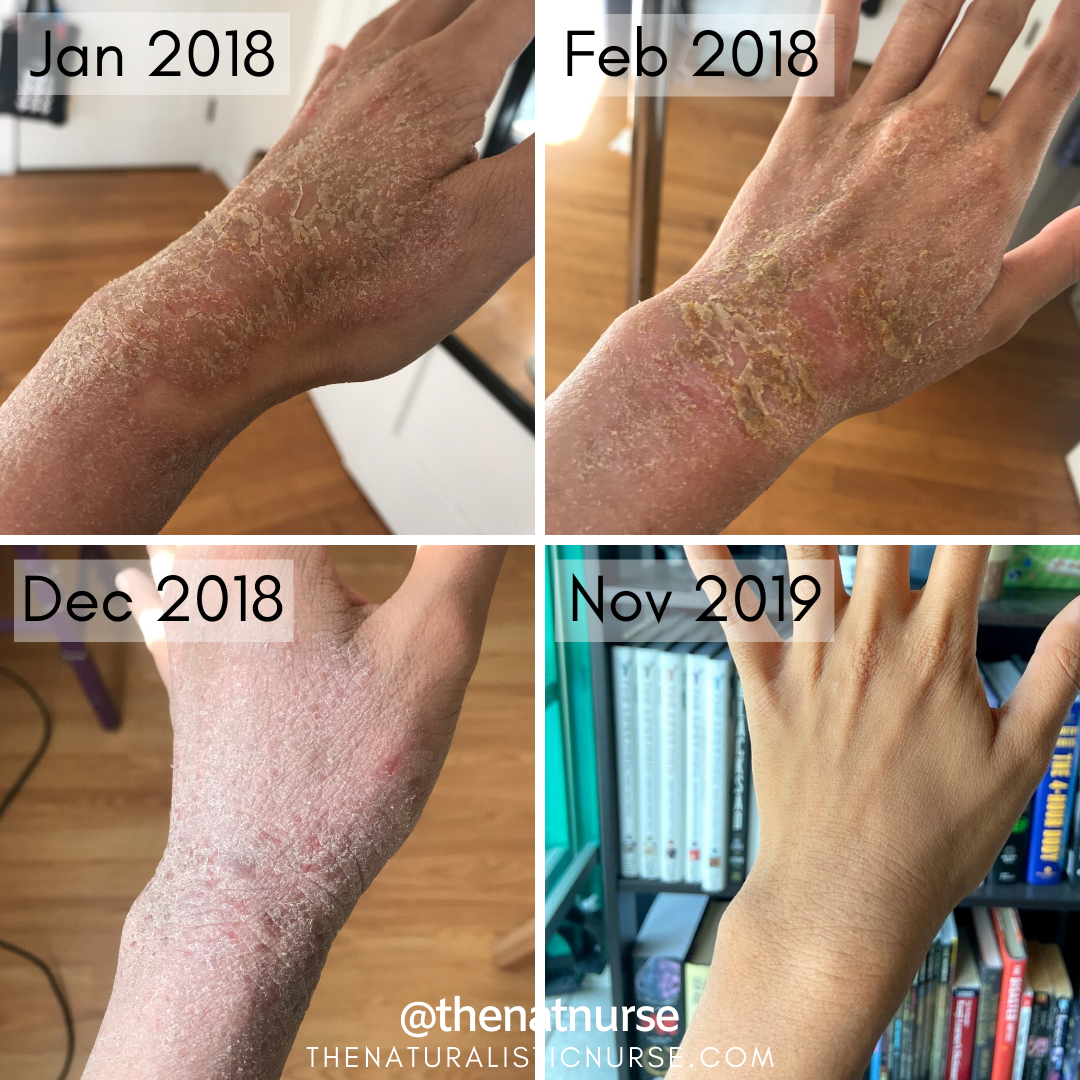This square image, measuring approximately six by six inches, contains a grid of four smaller square photographs set indoors. The layout features two images on the top and two on the bottom. The upper and one lower-left images are set against a light brown wooden floor, indicating the same room, while the lower-right image features a backdrop of metal shelving with books, suggesting a different location. Each photograph displays the left forearm and hand of a Caucasian individual afflicted with what appears to be psoriasis, characterized by thick brownish scales and red, irritated skin. The images document the progression and healing of the skin condition over time: January 2018 and February 2018 at the top, December 2018 at the bottom left, and a fully healed hand in November 2019 at the bottom right. The top left corner of each photo features a white square with black print denoting the date. The center bottom of the overall image displays text in white: "© thenatnurse" and beneath it, "thenaturalisticnurse.com."